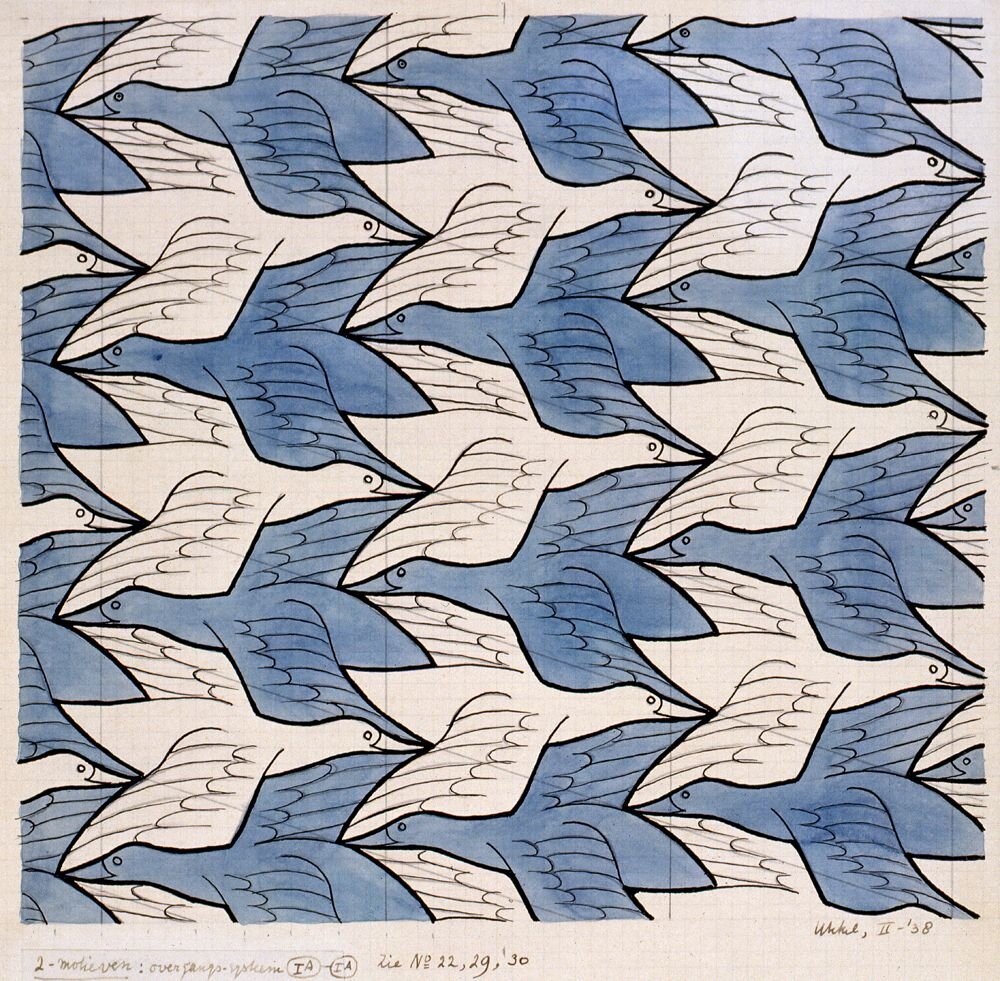The image depicts a carefully crafted tessellation artwork, showcasing an intricate repeating pattern of birds that bear a close resemblance to ducks or geese. The arrangement features rows of birds, with blue ones facing left and white ones facing right, forming a seamless interlocking design similar to puzzle pieces. Each bird, seen in profile, clearly displays its side and one visible eye, as well as detailed feather patterns on the wingspan. The precision of the image is highlighted by visible pencil lines used to perfect the geometry. Handwritten notes at the bottom of the image include partially readable text and numbers, such as "IA, IA" circled, a possible "22," "2G," and "30," followed by what appears to be a signature and "2-38." The artwork is professionally executed, with no gaps or holes in the tessellation, indicating a high level of craftsmanship.